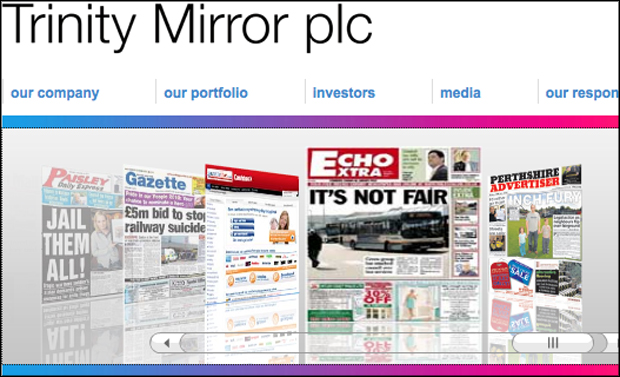This image displays a webpage interface primarily showcasing various magazine or newspaper covers. The top of the page prominently features the text "Trinity Mirror PLC." Below this, there is a navigation menu with sections labeled: "Our Company," "Portfolio," "Investors," "Media," and a partially obscured section labeled "Our Respond." 

A colorful gradient bar transitioning from blue to red spans the width of the page beneath the navigation menu. Below this gradient bar, there is an image displaying five vibrant newspaper covers. The titles of these covers include "Paisley Daily Express," "The Gazette," "Echo Extra," "Perthshire Advertiser," and one other title that is not clearly readable. 

At the bottom of the image, a small scroll wheel icon is visible, suggesting interactivity or further content exploration. The covers are colorful and reminiscent of celebrity gossip magazines, with various bold headlines and vivid imagery. Another gradient bar, similar to the one above the image, is placed below the picture, adding a symmetrical design element to the page.